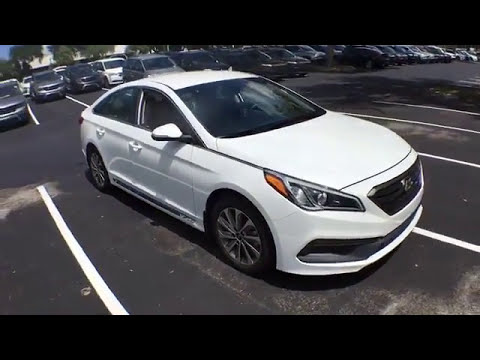The photograph captures a white four-door sedan parked slightly crooked in a designated space within a parking lot. The left front tire is almost touching the stripe, while the right front corner is angled away from the other stripe. Surrounding the car, the parking lot is marked with white lines and features multiple rows of parked vehicles, most of which are either white, gray, or black and are backed into the spaces. The lot's surface is a dark black tar, marred by stains and dirt of varying brown shades. In the background, there are visible tree lines and industrial-type buildings in the far distance, suggesting a city setting. The lighting is bright, indicating the photo was taken on a clear, sunny day. Additionally, there are some empty parking spots nearby, especially adjacent to the crookedly parked sedan. The sedan itself has clear headlights with an orange section, emphasizing its central position in the scene.